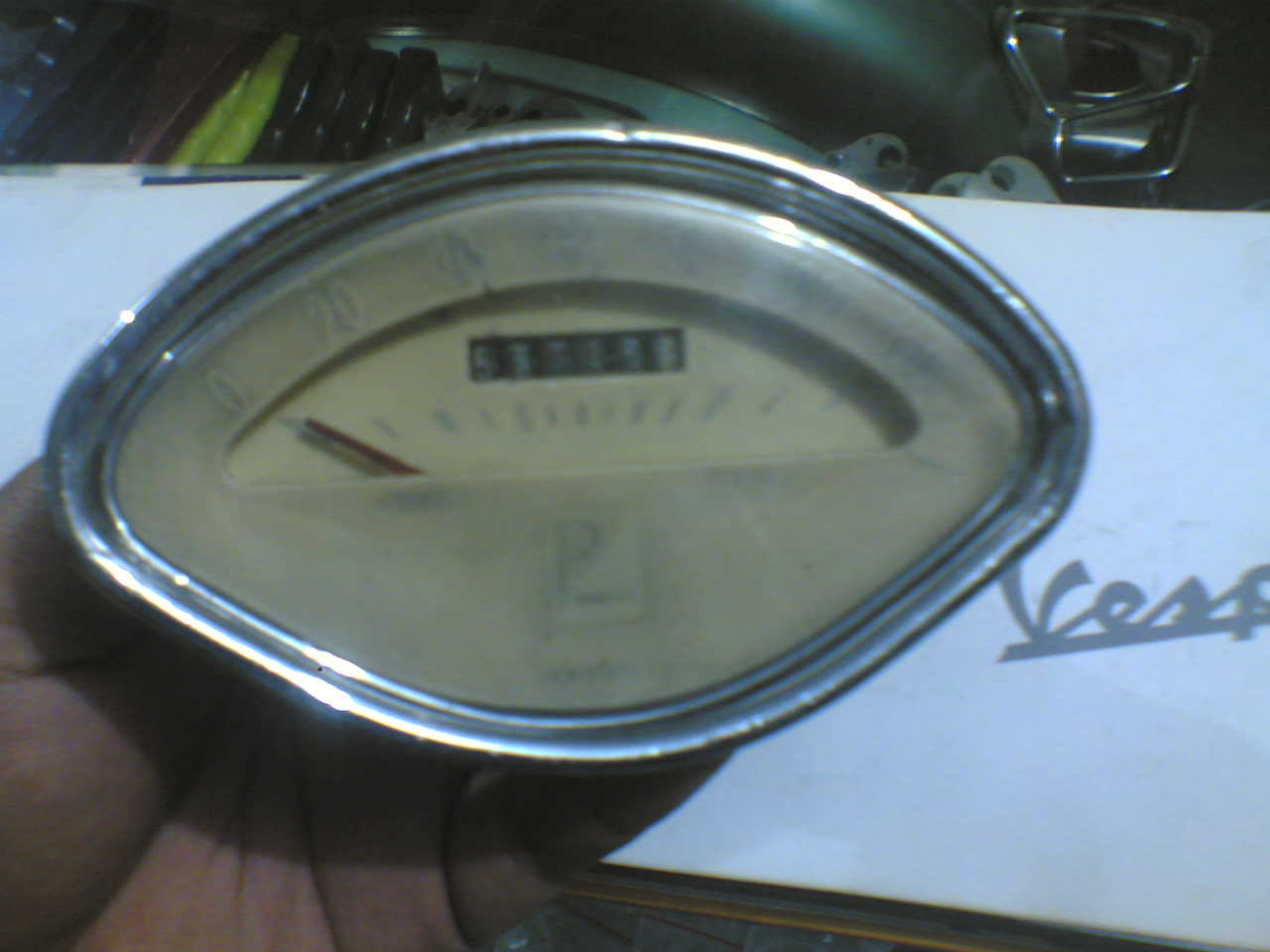A man holds an oblong-shaped odometer, resembling the shape of an eye with its slightly elongated bottom, close to the camera. The odometer is housed in a shiny metal case with a glass cover, giving it a vintage look. The cream-colored face of the odometer appears worn and a bit dirty from age. Though the exact mileage is unreadable due to the photo's blur, the odometer's display shows white numbers on a black background. A red needle points to zero, surrounded by grey dashes marking intervals, with numbers indicated from 20 onwards. Beneath the blurred numbers, the word "VESPA" is faintly visible in grey letters against a white backdrop. The background showcases parts of the VESPA motor in black, accompanied by visible yellow tubing, adding to the scene’s mechanical ambiance.